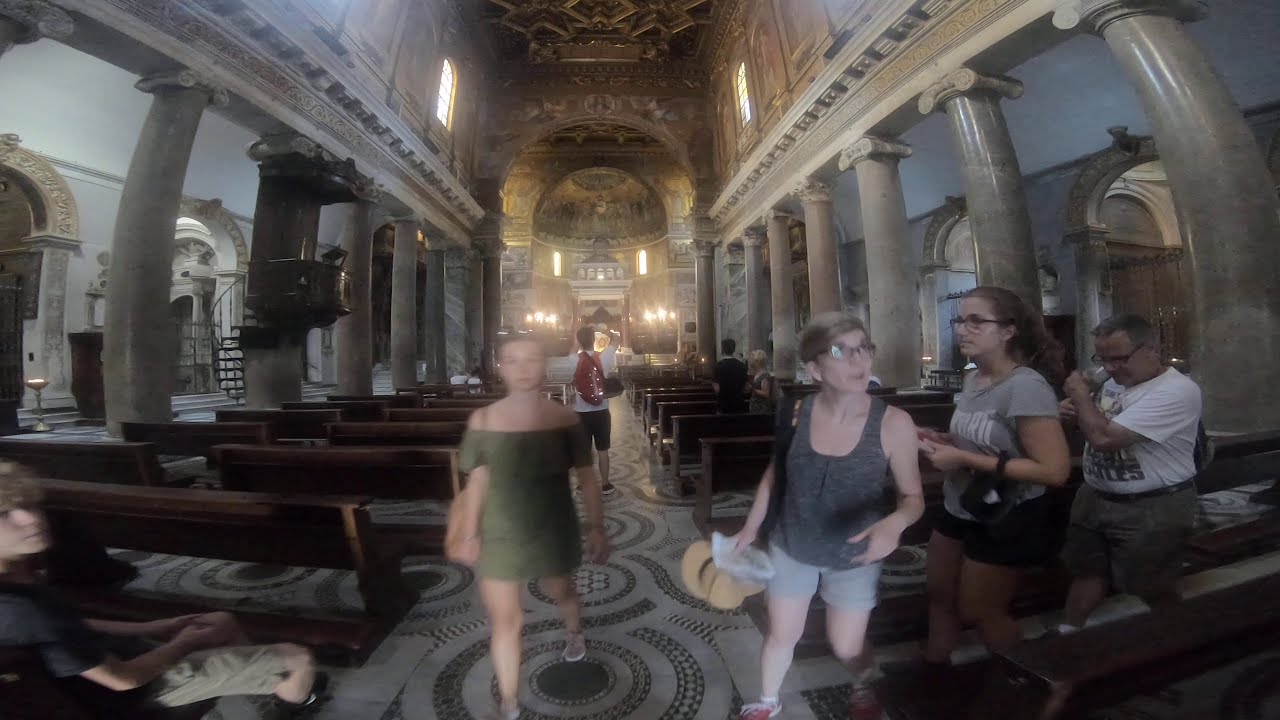The photograph captures a vibrant scene inside an impressive cathedral, possibly set in Europe, showcasing its grand architecture and lively ambiance. The cathedral features tall marble pillars reminiscent of Greek designs and intricate marble floors with swirling circular patterns. On either side of the central aisle, there are rows of brown wooden pews under majestic stone archways, leading up to a ceiling adorned with elaborate artwork.

Prominently in the foreground, a woman in a green sundress walks toward the camera, sporting white sandals and a purse on her shoulder. Behind her, a man with a red backpack, white shirt, black shorts, and black tennis shoes raises his arms, seemingly photographing the cathedral’s ornate ceiling. To the woman’s right, a trio, consisting of two women and a man, appears to leave the pews. One of the women wears a black sleeveless top and light blue jean shorts while holding a straw hat, the other has on a grey T-shirt with large writing, black shorts, and glasses, and the man is in a white shirt and dark shorts.

In the background, additional visitors can be seen exploring the cathedral, including a man and a woman with their backs to the camera. The architectural elements, including a wrought-iron staircase spiraling to the ceiling and a canopy area possibly meant for ceremonies, add to the grandeur of the setting. The overall scene reflects the bustling and awe-inspiring experience of visiting such a historic and culturally significant landmark.